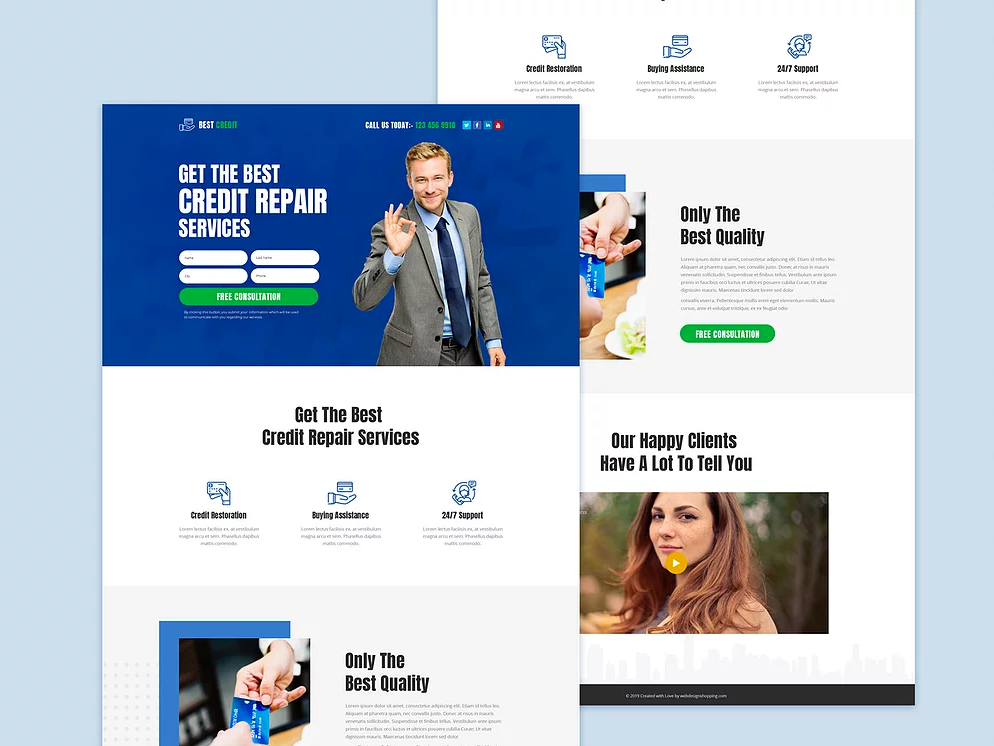The image displays a superimposed view of two web pages related to credit repair services. The front page prominently features a green button labeled "Free Consultation." Next to it, a smiling man with blonde hair, wearing a suit and tie, gestures with an "OK" sign using his thumb and index finger, while his other three fingers are extended. Above this, the text reads "Get the Best Credit Repair Services." Additional offerings listed include "Credit Restoration," "Buying Assistance," and "24/7 Support." Below these services is a statement in black text: "Only the Best Quality." The second page, slightly visible in the background, provides more details under the heading "Our Happy Clients Have a Lot to Tell You" and includes a thumbnail for a video of client testimonials.